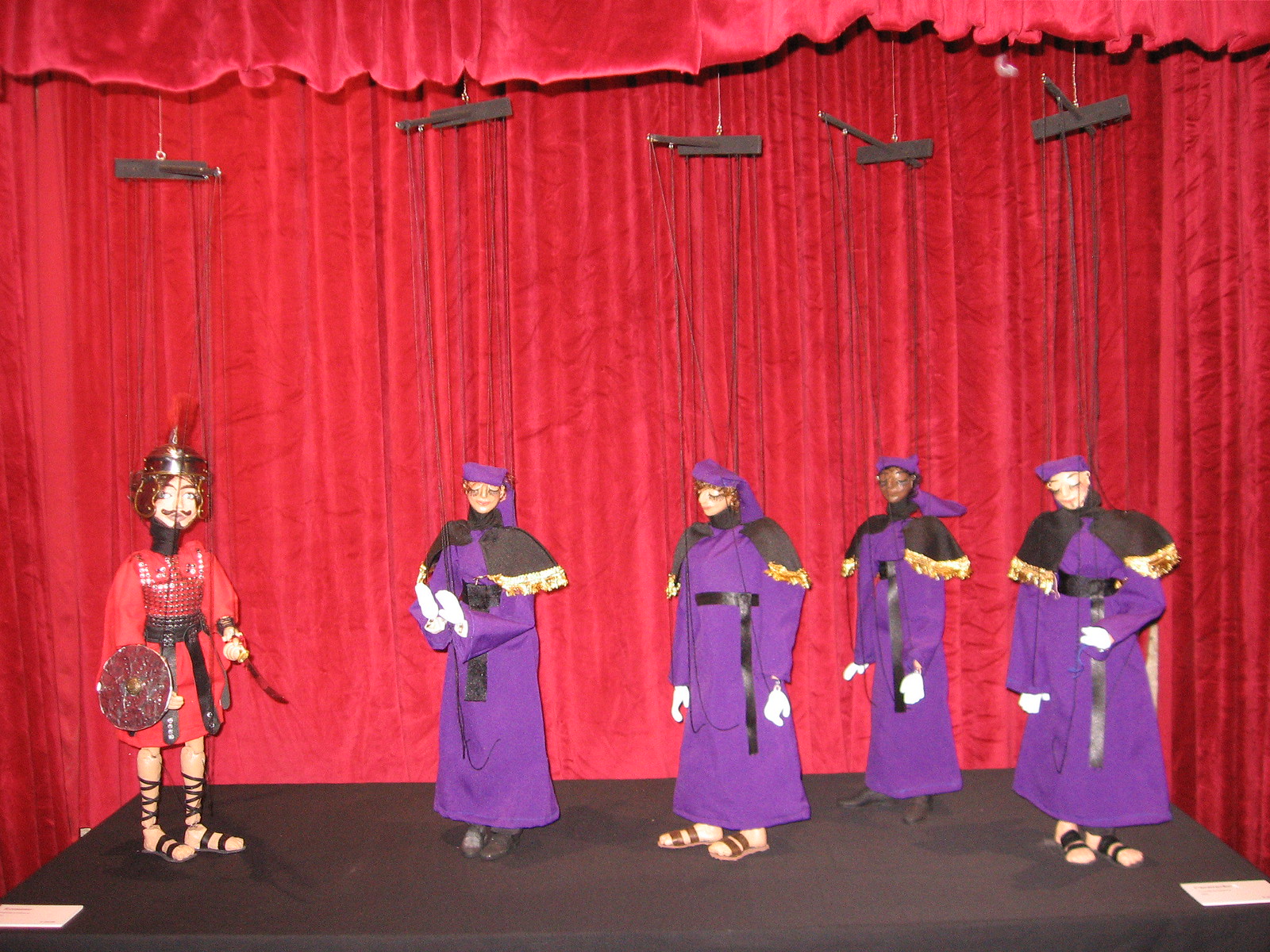The image depicts a vivid puppet scene set against a backdrop of rich, velvety red curtains. Arrayed on a black fabric-covered stage, five intricately-detailed puppets rule the display. The central puppet, a regal male figure, commands attention in a red medieval outfit adorned with a crown and equipped with a sword and a red shield. His attire includes gladiator-style sandals and a darker-toned belt. Suspended by black or dark brown strings from a brown rectangular bar above, his strings are meticulously visible.

Flanking this knightly puppet are four female puppets, each garbed in long, flowing purple robes with black and gold highlights, reminiscent of ecclesiastical attire. White gloves cover their hands, adding to their dignified appearance. They share the same detailed sandals, varying in black and brown hues, and their heads are covered with matching purple headpieces. All five puppets, painstakingly crafted and suspended by strings, stand poised on the black fabric stage, framed by the opulent red curtain backdrop, evoking the traditional charm and grandeur of a classical puppet theatre.